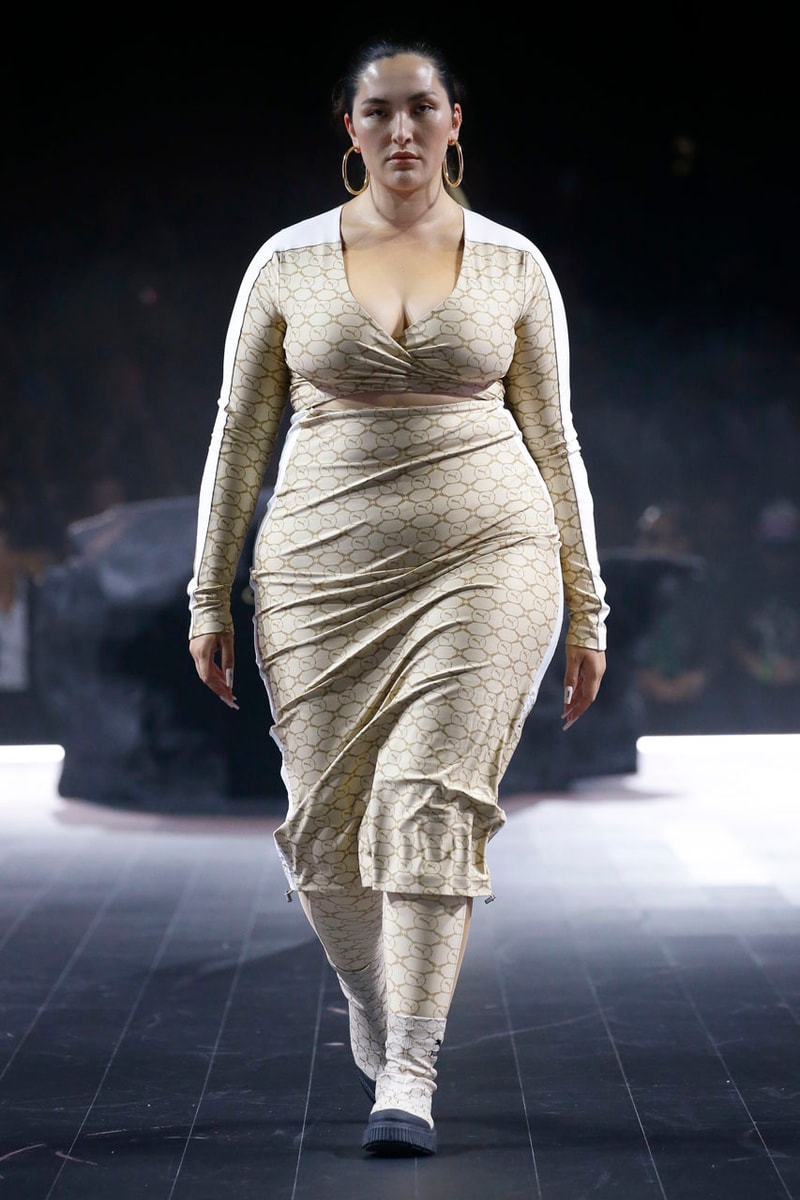The image depicts a curvy, plus-size model confidently striding down a runway. She is dressed in a beige, form-fitting dress adorned with golden geometric patterns, and the dress extends below her knees. Her attire includes long sleeves and a neckline that reveals a bit of cleavage. Complementing her outfit, she wears matching white boots with blue soles, maintaining the geometric pattern motif. She accessorizes with oversized hoop earrings and sports long fingernails. The model has dark hair, and her expression is serious, devoid of a smile. Despite the background being blurry, it is discernible that there is an audience watching her, adding to the atmosphere of a fashion show. The entire setting, including the stage and floor, features blue tones with a checkerboard pattern.